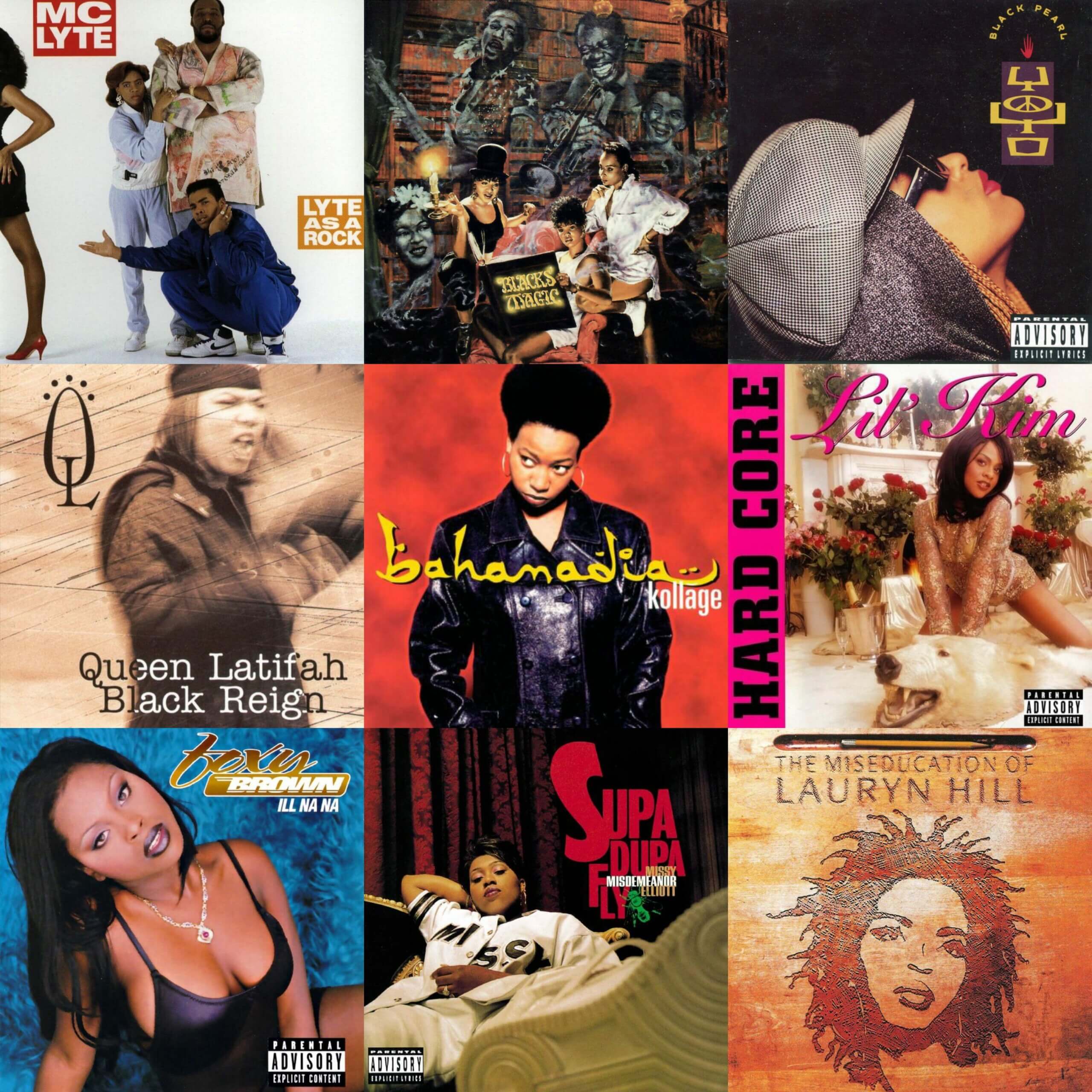This image is a collage of nine album covers, each by prominent African-American female artists, arranged in a three-by-three grid. The top left corner features MC Lyte's "Lyte as a Rock," showcasing a man in a tracksuit squatting, with a taller man behind him and a woman beside him. Next to it is Salt-N-Pepa's "Blacks' Magic," which depicts three women: one seated with an open book and two standing beside her, against a mural background. The top right is Yo-Yo's "Black Pearl," presenting the artist with her head tilted back, wearing a gray hat and sunglasses on a black background.

The middle row begins with Queen Latifah's "Black Reign," featuring the artist against a brown backdrop. The center cover is Bahamadia's "Kollage," showing her with a big afro, a red background, and a leather jacket. To the right is Lil' Kim's "Hardcore," where she poses provocatively on a bear skin rug, surrounded by a pink border.

The bottom row starts with Foxy Brown's "Ill Na Na," which has her in a little black dress against a blue background. Next is Missy Elliott's "Supa Dupa Fly," depicting her reclining on a chair or couch. The final album in the bottom right is Lauryn Hill's "The Miseducation of Lauryn Hill," illustrated with a drawn image of her face on a brown background.

The diverse colors and unique styles of each cover reflect the individual flair of the artists while collectively celebrating the significant contributions of black female musicians in the industry.